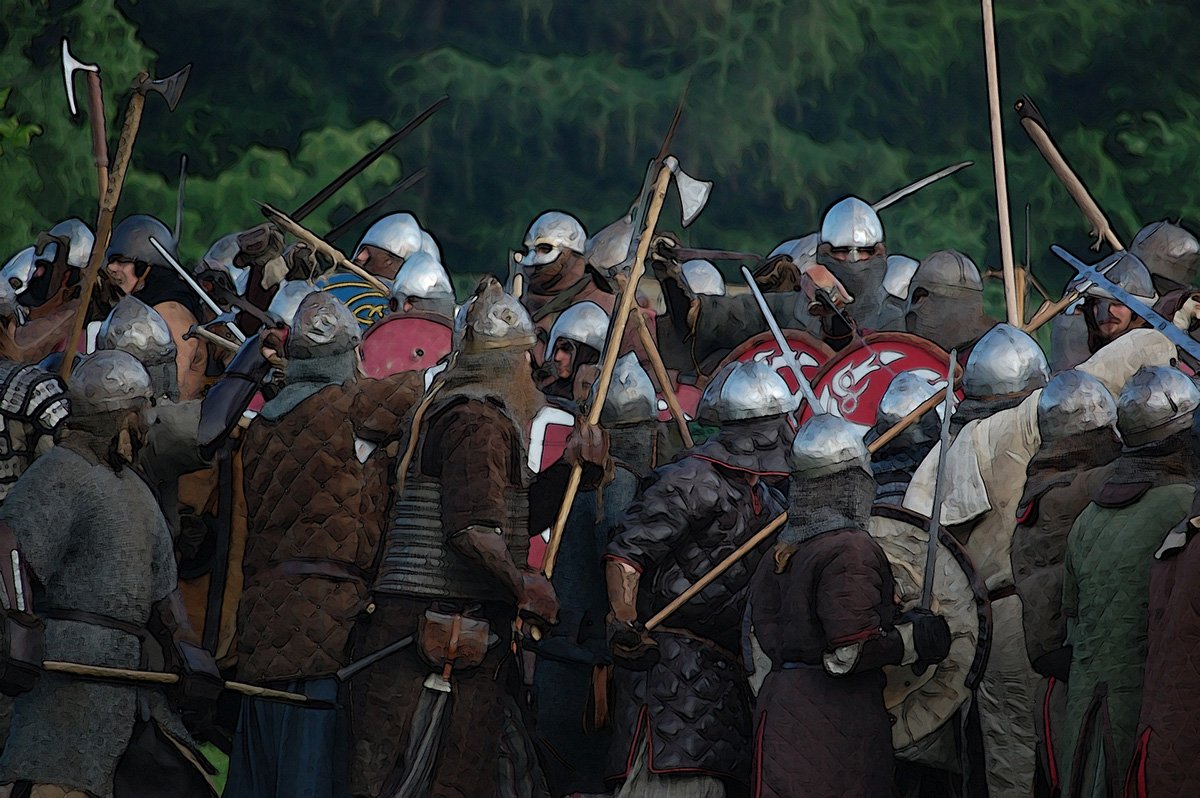The image depicts a stylized, animated scene resembling a medieval battle, set against a backdrop of lush green trees. The foreground is filled with diverse warriors clad in various medieval armor, including chainmail and padded cloth tunics. Each soldier sports a distinct shiny metal helmet, some featuring face protection that ranges from full masks to minimal coverage. They wield a variety of weapons such as swords and long-handled axes, and some carry shields adorned with red and white designs. The soldiers' attire is mostly composed of browns, grays, and reds, complemented by small leather bags. The image has a unique visual effect, possibly resembling cell shading or a watercolor painting, giving it a slightly smudged, artistic quality. The scene captures the intensity of battle, with warriors grouped and facing multiple directions, suggesting dynamic movement and action.